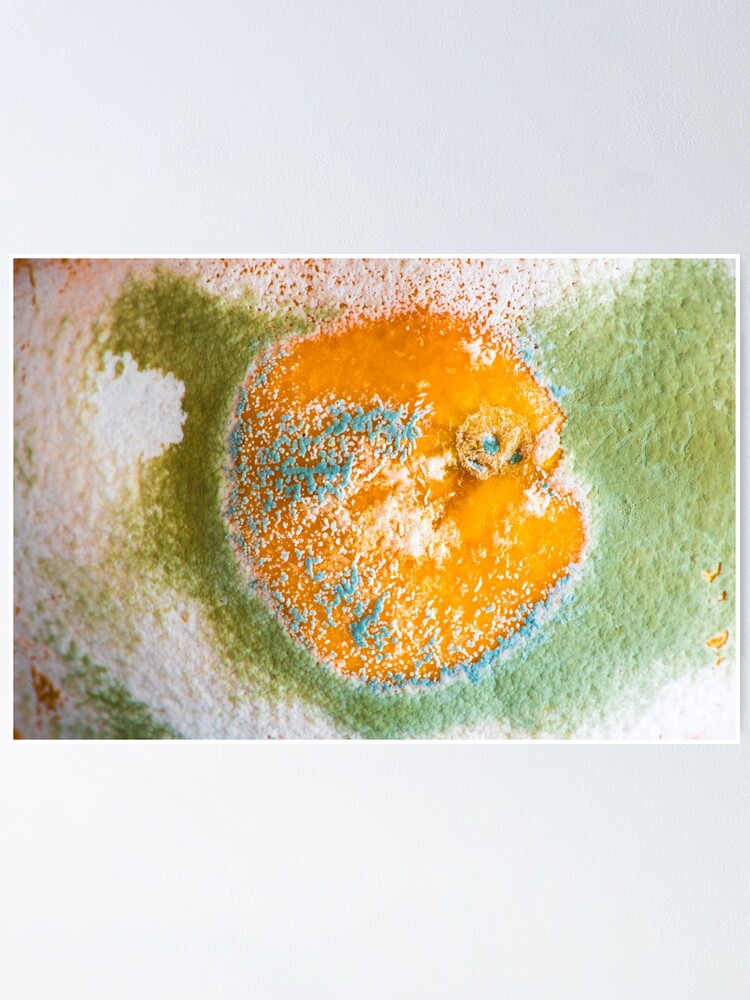The image depicts a close-up of a severely moldy piece of fruit, potentially a cantaloupe or an orange. Dominating the center is a bright orange circle, characteristic of an orange peel with the distinctive eye piece indicative of where it once attached to the tree. This circle is surrounded by a textured, moldy surface showcasing patches of vivid green and white mold. There are also splotches of blue mold distributed across the orange surface, resembling the rough, cracked texture of plaster or aged leather. The irregular mold patterns reveal bits of pink and dark red on the top left, with an intricate mix of white, dark red, and green in the bottom left; the bottom right remains predominantly white, while the top right corner is entirely green. The fruit is framed with a thin white border, set against a dark gray background, giving the entire composition an eerie, close-up microscopic appearance.